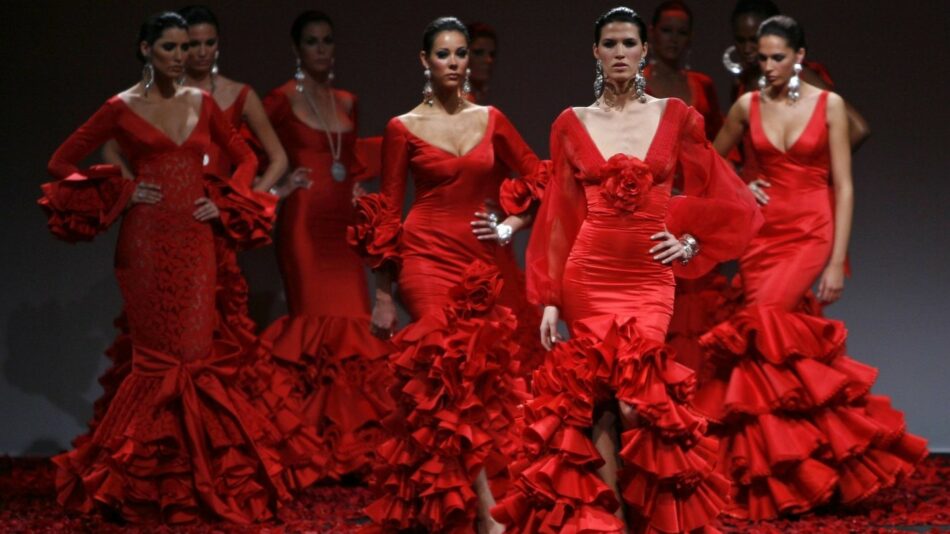In an indoor setting lit by studio lights, a group of nine women is posed on a fashion runway, dressed in striking, form-fitting, cherry-red mermaid-style dresses that feature deep décolletage and end in tiers of ruffles. Their outfits vary subtly, with some dresses adorned with bows, ruffles, and rose floral decorations. The sleeves also differ, ranging from sleeveless to ruffled or poofy, gauzy designs. Each woman, either white, black, or medium-skinned, wears her dark brunette hair tightly pulled back, except for one black-skinned woman and one blonde in the back row. They all sport large, oversized earrings, and a few add large silver necklaces to their ensemble. Striking a poised and confident stance, most of the women have one hand on their hip, suggesting a fashion show or pageant, with a backdrop of dimmed gray and black emphasizing their bold, smoky eye makeup and the elegance of their coordinated attire.